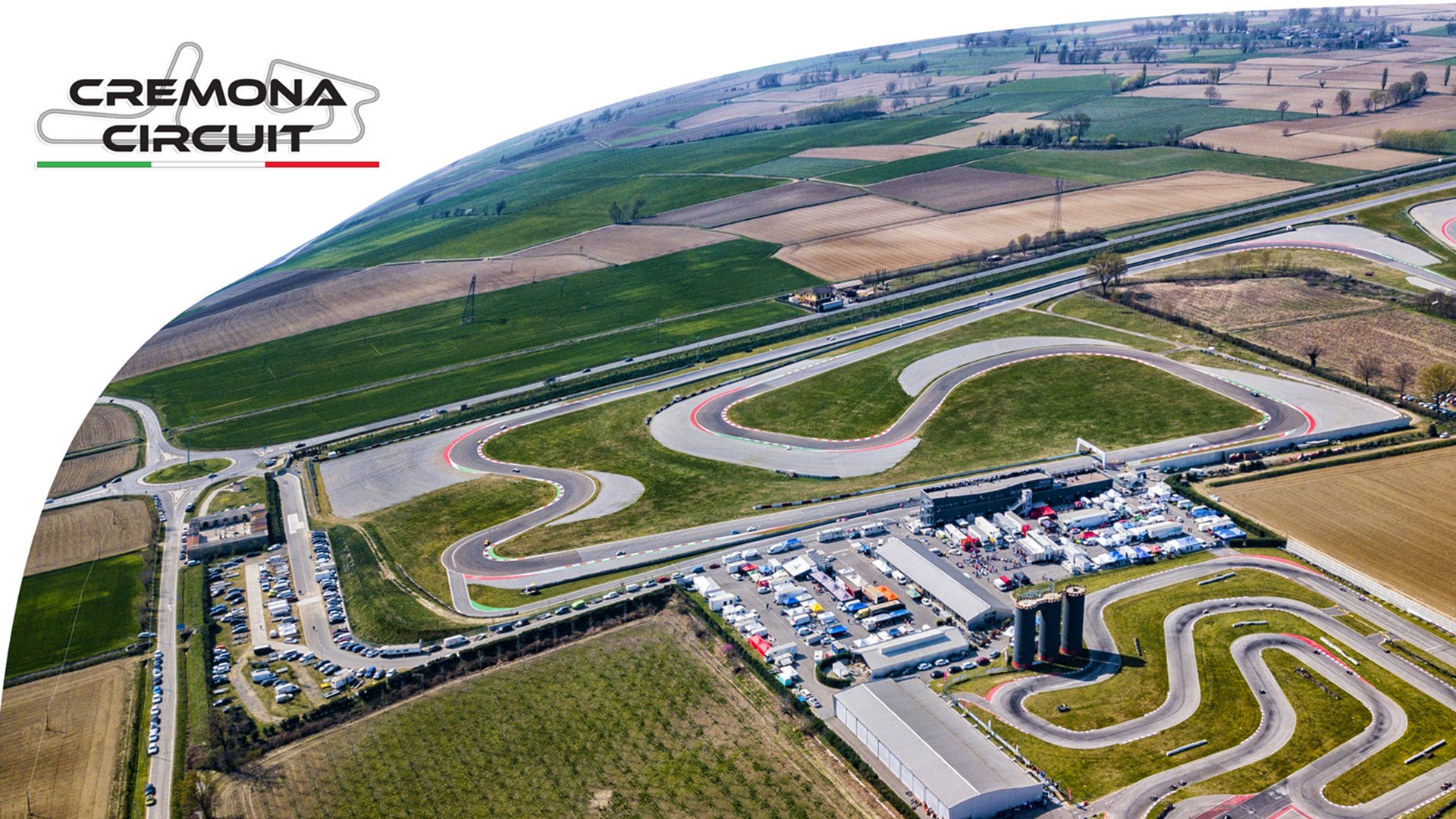This aerial photograph showcases an expansive industrial park, centrally featuring prominent silos and a distinct test track, all bearing the label "Cremona Circuit" in white text with the colors green, white, and red underneath. The park itself is dotted with many cars spread across various parking lots, underscoring its active use. A network of driveway connections links clusters of buildings, emphasizing the park's organized structural layout. In the background, another larger track suggests additional testing or recreational facilities. Surrounding the industrial area, extensive green and brown pastures hint at ongoing farming activities, with the uniform rows of crops and the beige-tan fields further framing the scene. Trees line the edges of some fields, adding a touch of natural separation between areas.